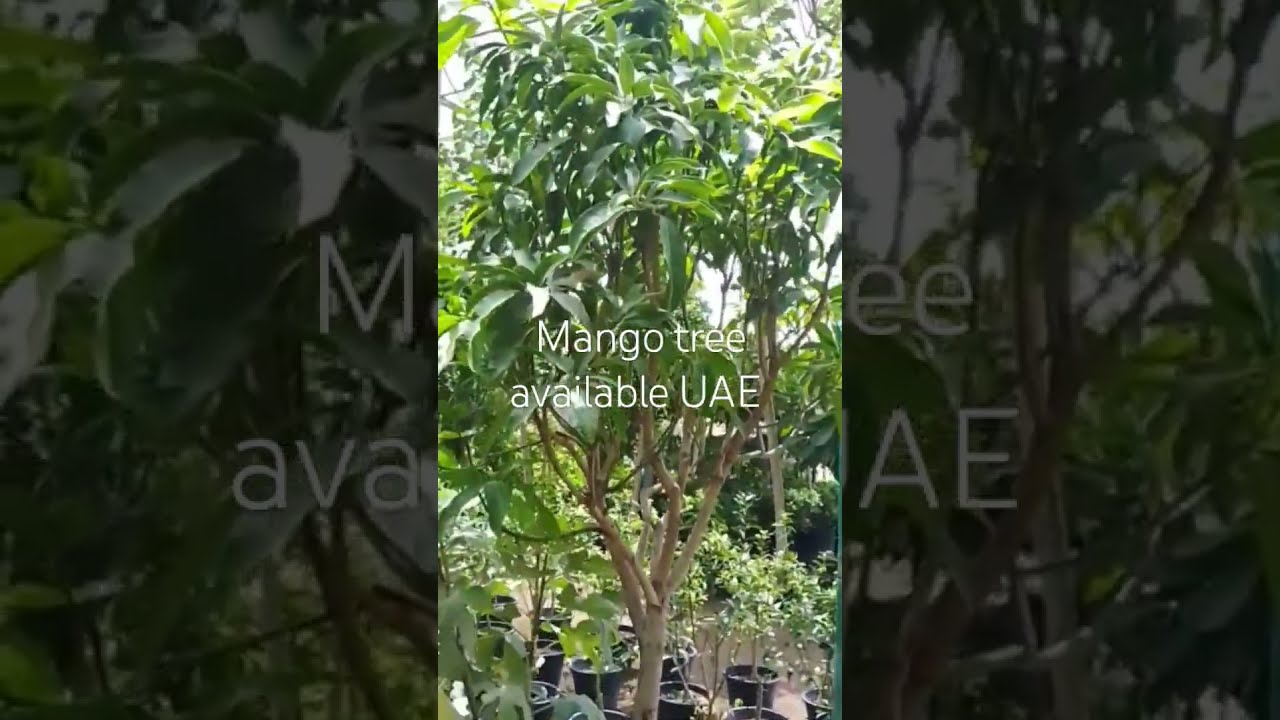The horizontal rectangular image features a prominent central vertical rectangle in vibrant color that showcases a mango tree. The tree, with its light brown trunk, stretches out its branches covered in lush, large green leaves, extending towards a bright sky. Beneath the tree, rows of black potted plants, each containing young trees, are visible. The image has white text at its center, reading "Mango Tree Available, UAE," with the lines of text neatly centered on top of one another.

Flanking this central colored image are two faded, darker close-up sections of the tree, creating a frame-like background. These sections, darker and more shadowed, display fragments of the text from the center, with parts of the words "Mango Tree Available, UAE" visible on both the left and right sides. The entire composition highlights the vibrant mango tree in the middle while providing a mirrored, subdued perspective on either side, enhancing the focal point of the central tree.